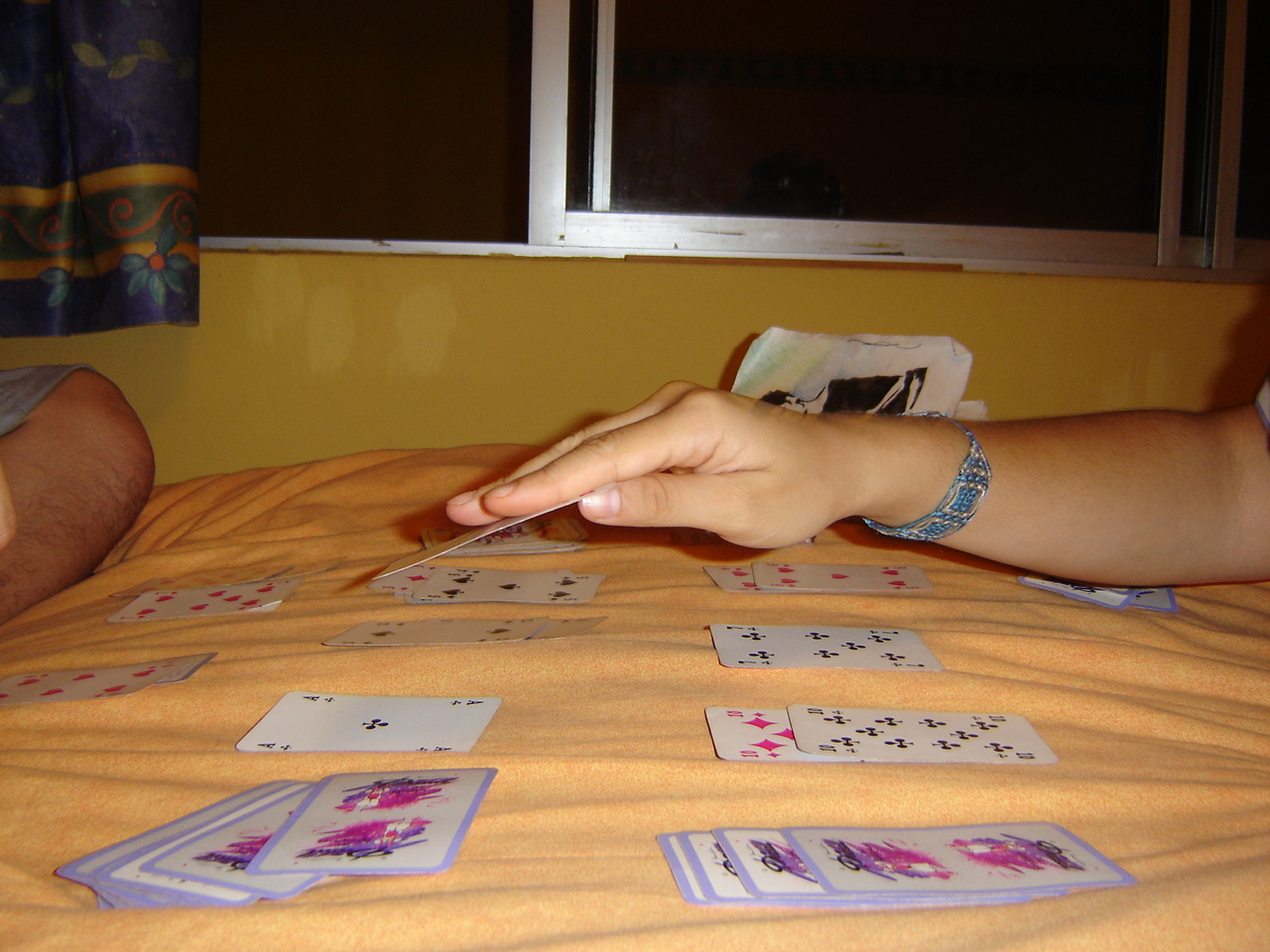In this nighttime photograph, an individual is engrossed in a card game, seemingly seated on a plush comforter that tops a bed. The scene is illuminated subtly, with another person’s knee and knuckle slightly visible on the left, suggesting their potential involvement or observation. The individual on the right, likely a female, has neatly groomed fingernails and is captured in the act of placing a card towards the center, hinting at a game of solitaire. Her forearm is adorned with a striking bracelet that appears to feature turquoise stones. Behind her, through a glass window with a silver metal frame that is slid open, the darkness of the outside night is evident, enhancing the intimate indoor setting. The upper left corner outside reveals leaves, seemingly part of a drape, fluttering near the window. The soft surface beneath the game, resembling a comforter's bowed top, cradles the colorful and intricately designed card backs. Adjacent to the woman's arm, a small stack of bags or papers lends a casual, relaxed atmosphere to the space.